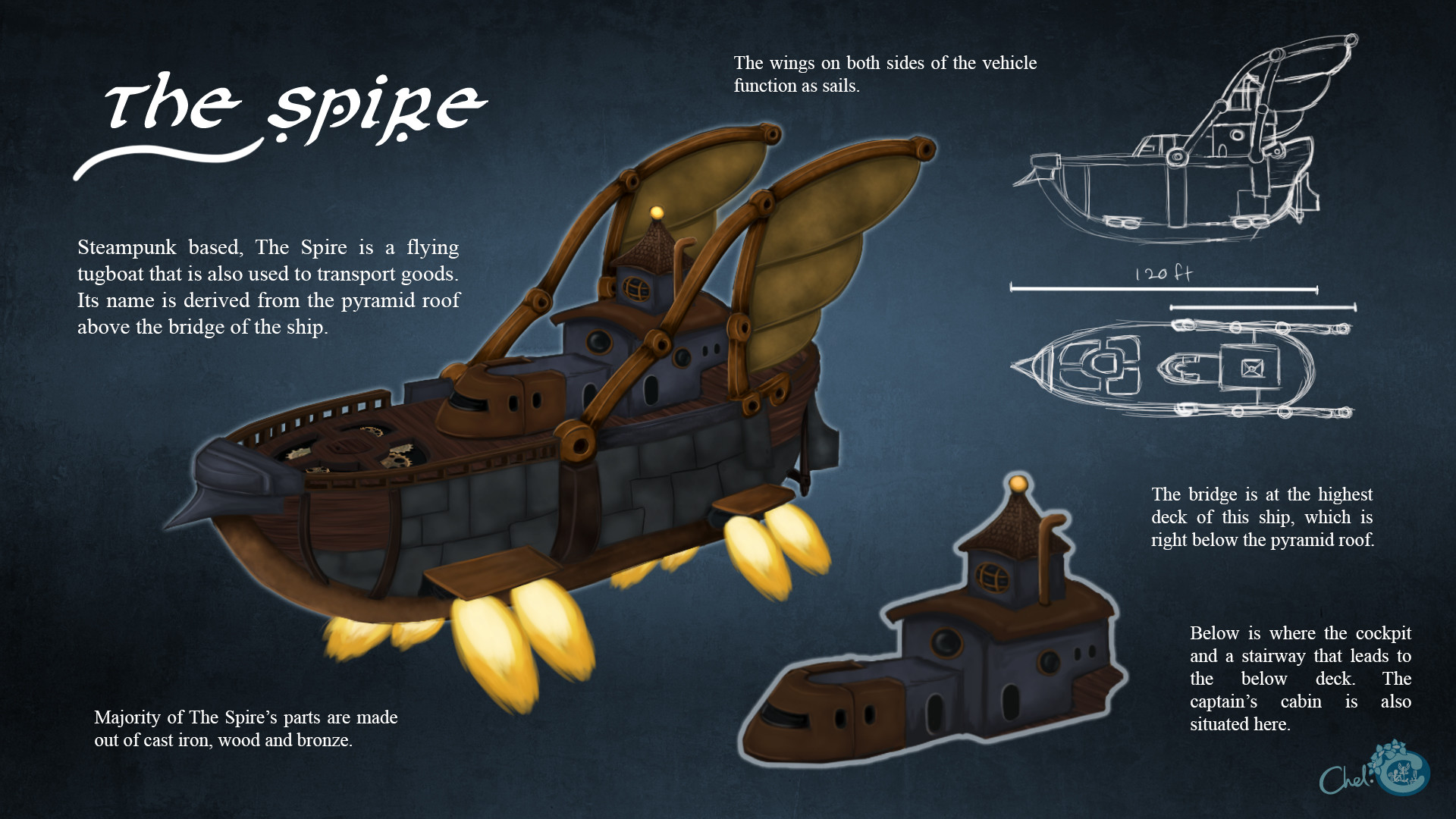This is an intricately detailed informational poster with a steampunk theme, set against a dark blue background. Central to the poster is a brown flying tugboat named "The Spire," designed with a pyramid-shaped roof above the bridge, which inspired its name. The vessel features wing-like sails on either side and is depicted in both a side profile and a top view in white outline drawings. The bridge is located at the highest deck, just below the pyramid roof. White text around the poster provides descriptions, noting that "The Spire" is used to transport goods and highlighting various elements like the sails functioning as wings and the engine-based propellers. The colors utilized in the poster are black, white, dark blue, brown, light brown, gray, and yellow, giving it a rich, vintage aesthetic.